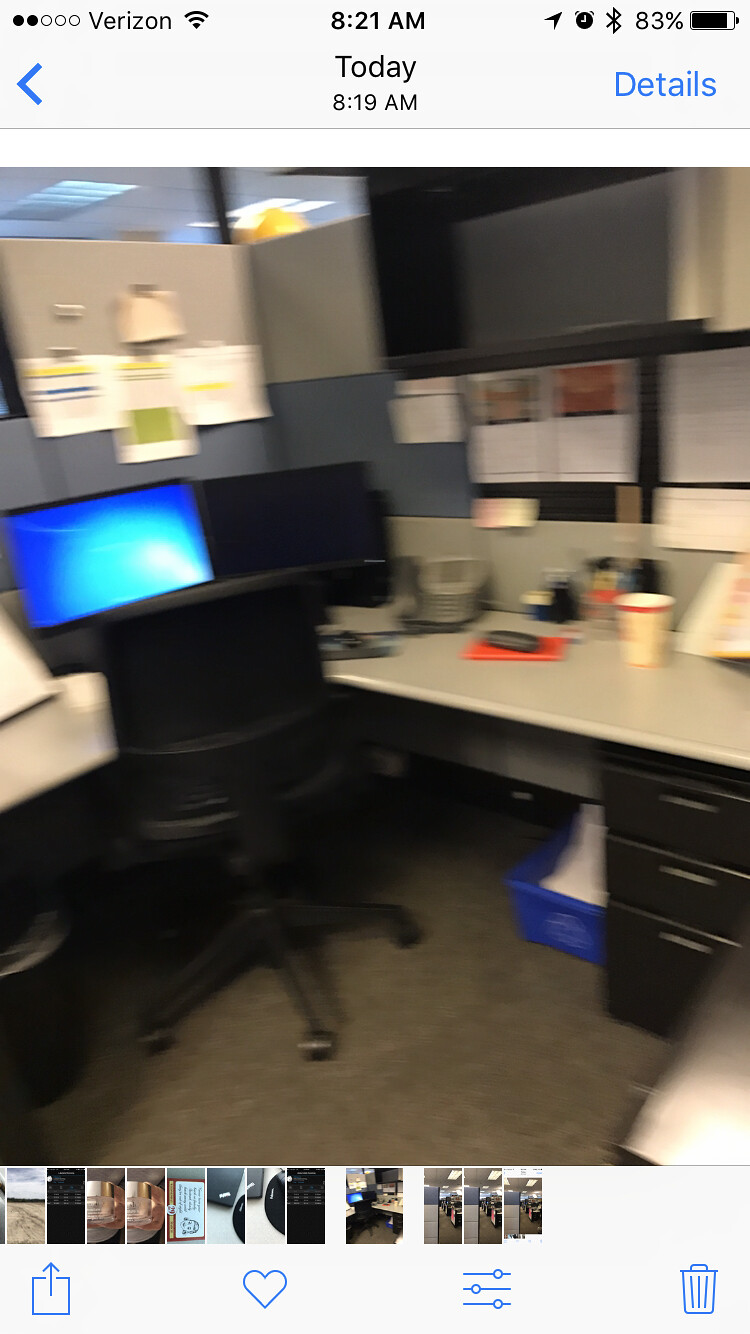A slightly blurry vertical photograph of an office cubicle captures a typical white-collar workspace. At the center of the image, an office chair is positioned with its back towards the viewer, tucked into the corner of an L-shaped white desk. The desk supports a desktop computer monitor displaying a blue screen, with a possible second monitor positioned to the right. Scattered across the desk are various office essentials, including a coffee cup and a standard office telephone. Below the right side of the desk, a blue recycling bin is visible, alongside a set of black pull-out drawers. The beige partition walls are adorned with items like calendars and notes, while additional storage units are mounted on top of the partitions. In the upper left corner of the image, the ceiling features standard acoustical tiles and recessed acoustic paneling, completing the quintessential office environment.